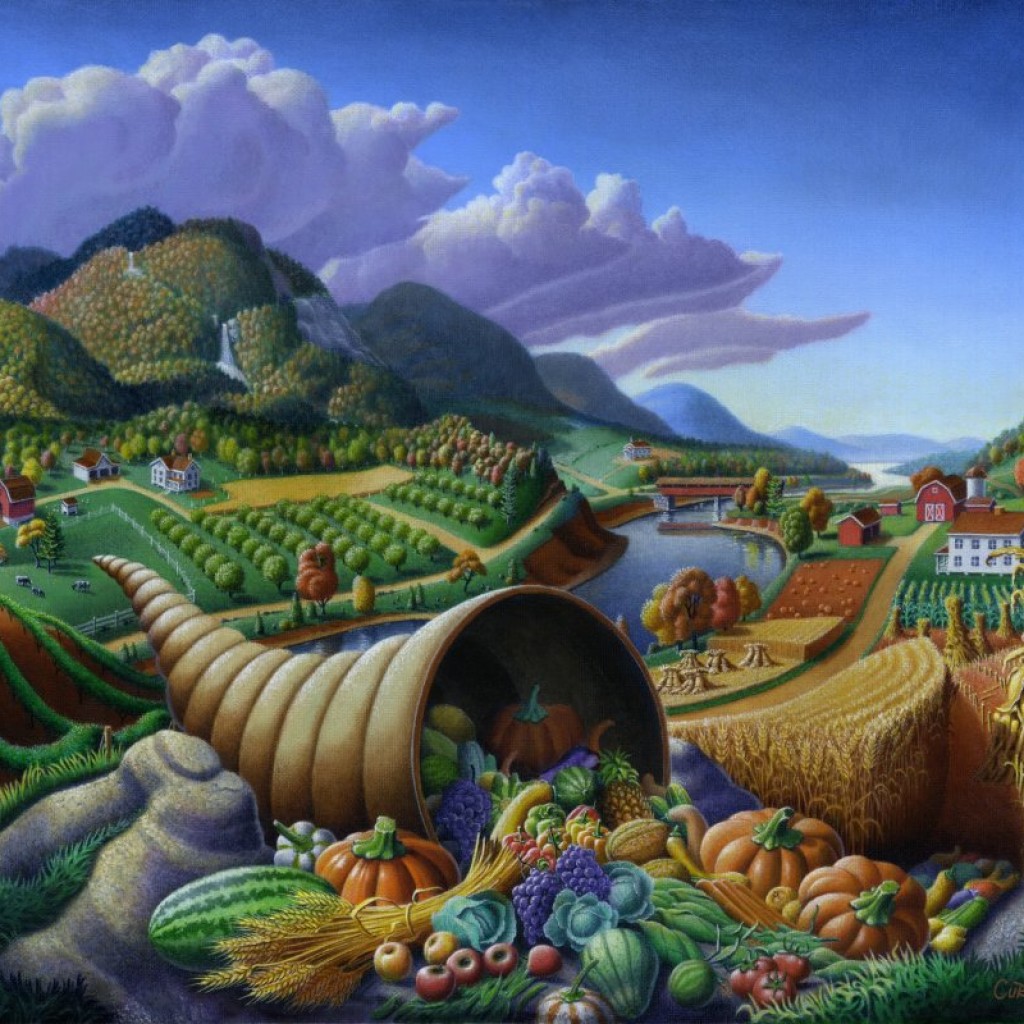This vibrant digital artwork, rendered in a fantasy-cartoon style, features a prominent tan cornucopia in the foreground, overflowing with a diverse array of fruits and vegetables, including orange pumpkins, red apples, green gourds, watermelons, corn, squash, wheat, radishes, tomatoes, pineapples, and grapes. The scene is set on a lush, colorful grassy area. Behind the cornucopia, the viewer is given an illustrated bird's-eye view of a storybook-like farming town.

To the right, plot sections of tan and rust-brown farmland are visible, with neatly planted crops and a distant red barn, complemented by a white house nearby. Meanwhile, on the left, the landscape transitions into high tree-topped hills adorned with fluffy clouds, gray at the bottom and white on top. These hills slope down towards a river that weaves gracefully through the valley, delineating the farming plots on either side.

Further into the distance, round trees border the hills, and a few houses are nestled among them. The sky above transitions beautifully from mid-tone to light blue, punctuated with purple-tinted clouds floating overhead. Completing the picturesque backdrop is the silhouette of a majestic mountain range, adding depth and grandeur to the enchanting scenery.